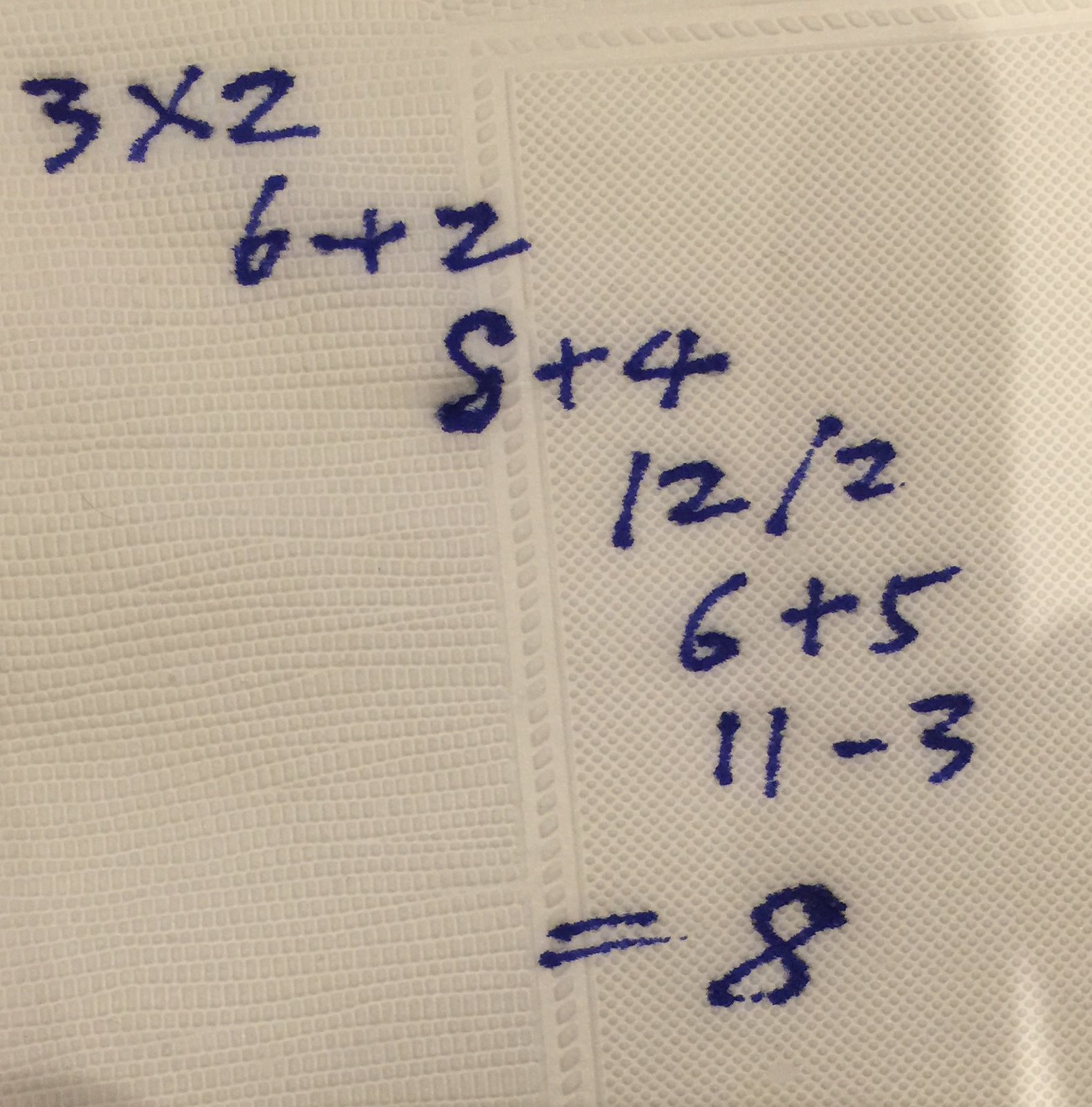This is an ultra-close-up image of a textured white napkin, revealing its intricate woven pattern. The napkin's fabric showcases a series of raised, small, square shapes arranged in a repetitive design. Overlaid on this textured background, someone has written a series of math problems using a blue fountain pen. The ink appears thick and somewhat smeared, characteristic of fountain pen usage rather than a ballpoint pen. 

At the top of the napkin, the number "3x2" is prominently displayed. Slightly below and to the right is "6+2". Following this, there is "8+4" also positioned to the right. Beneath these, "12/2" is written, followed by "6+5". Below that is the arithmetic problem "11-3". At the very bottom of the napkin, an "=" symbol is present, leading to the number "8" which features a noticeable ink blot on the upper right part of its curve, indicating excess ink from the pen.